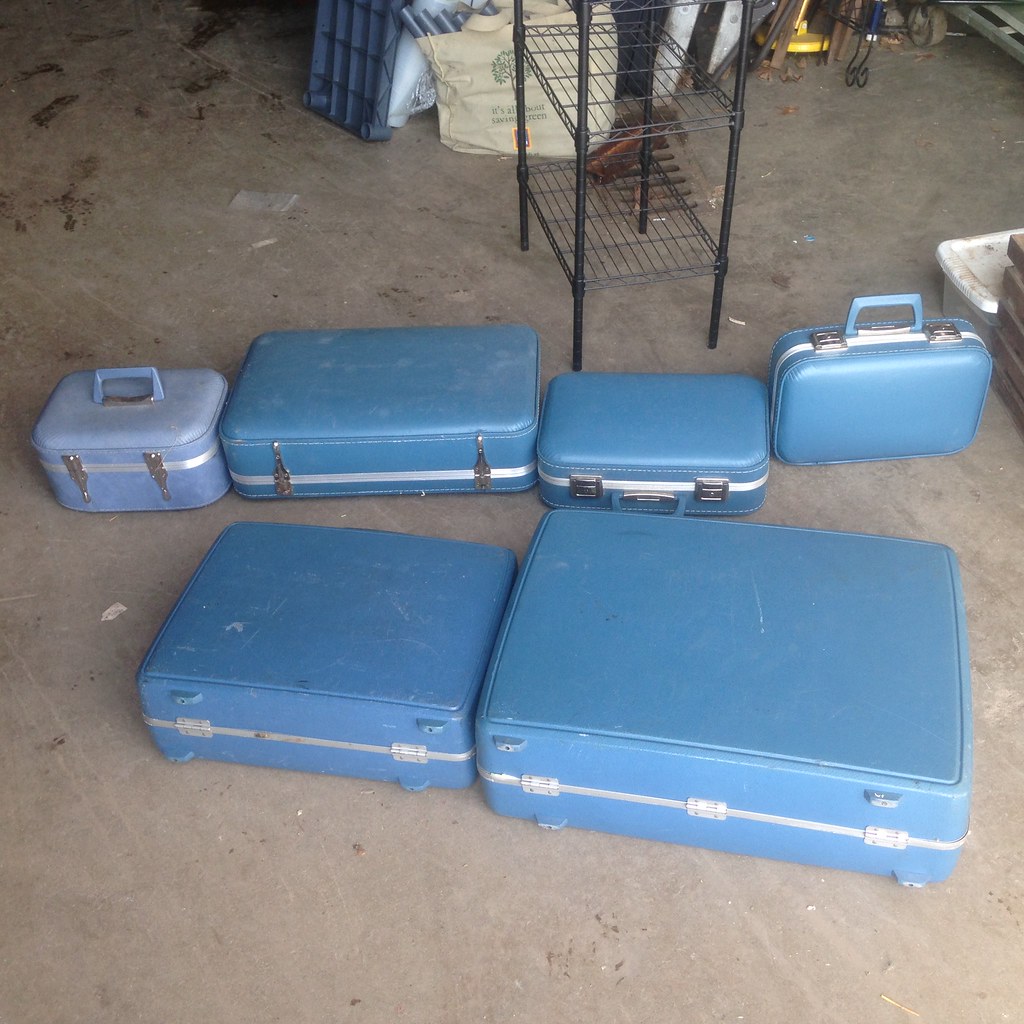This detailed photograph captures a collection of light blue suitcases arranged on a concrete floor, likely within a basement or storage warehouse setting. The suitcases, all featuring silver hinges and exhibiting signs of wear with scratches and dirt marks, evoke an old-fashioned style of travel luggage. The scene presents six suitcases in total, uniformly blue except for one lighter shade.

In the foreground, there are two large rectangular suitcases positioned horizontally on the floor. To the left, a light blue suitcase with silver hinges stands upright. The right foreground showcases a larger rectangular suitcase with silver hinges and a distinctive white line. Additionally, a small rectangular suitcase lies on its side nearby. On the far right, another small suitcase rests upright with a blue handle.

The background of the image reveals a metal rack filled with bags and other assorted items, contributing to the cluttered and utilitarian atmosphere. The ground beneath these suitcases appears to be concrete, adding to the raw, storage-like environment of the scene.